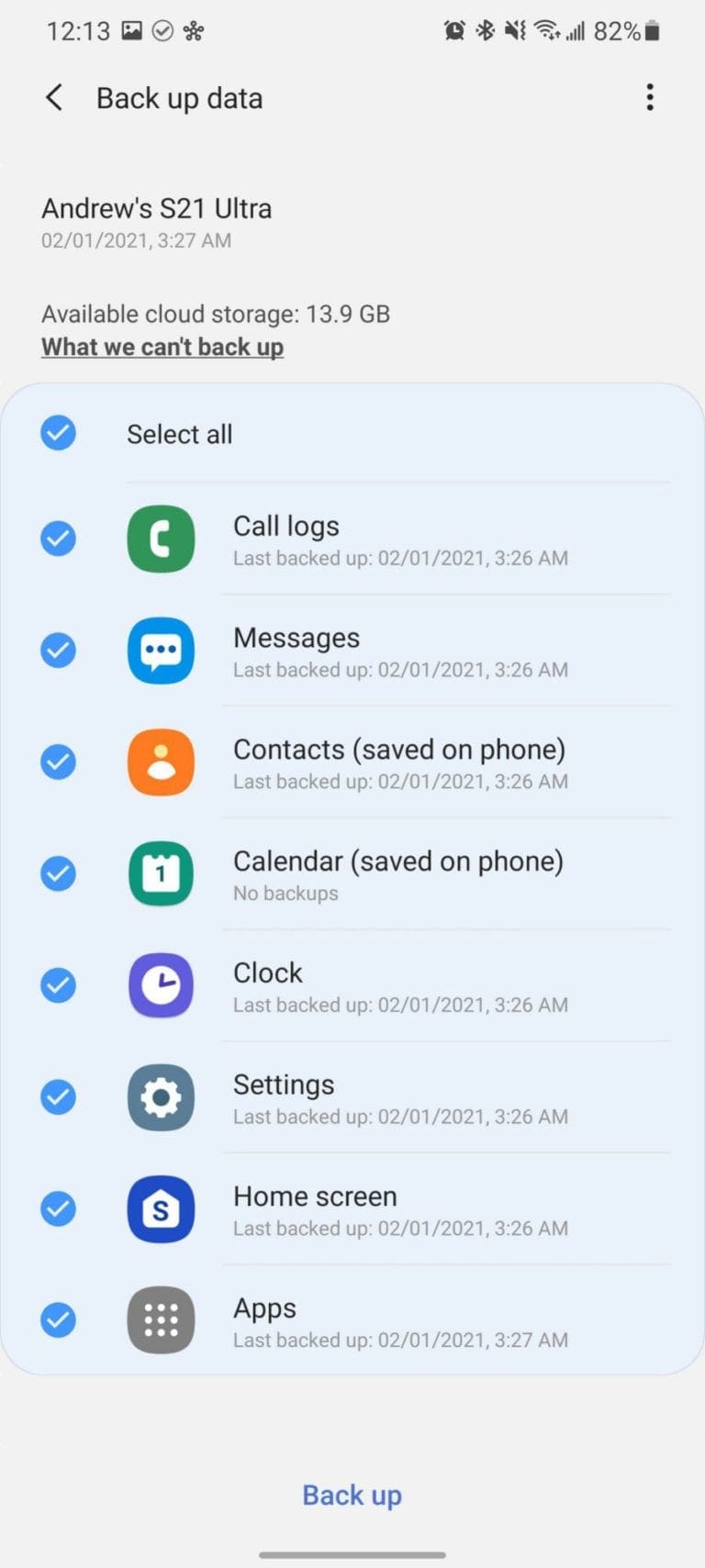Screenshot of an Android phone displaying the "Backup Data" settings screen. The notification bar at the top shows it is 12:13 PM, with a few notifications visible. The alarm clock is set, Bluetooth is connected, sound is muted, Wi-Fi and network signals are full, and the battery is at 82%. The device is identified as Andrew's Samsung Galaxy S21 Ultra. The date and time currently display as January 20, 2021, 3:27 AM. Available cloud storage is 13.9 GB. All backup options are selected, including call logs, messages, contacts, calendar, clock, settings, home screen, and apps, each represented with their respective icons. At the bottom, a blue "Backup" button indicates that Andrew is ready to initiate the backup process.